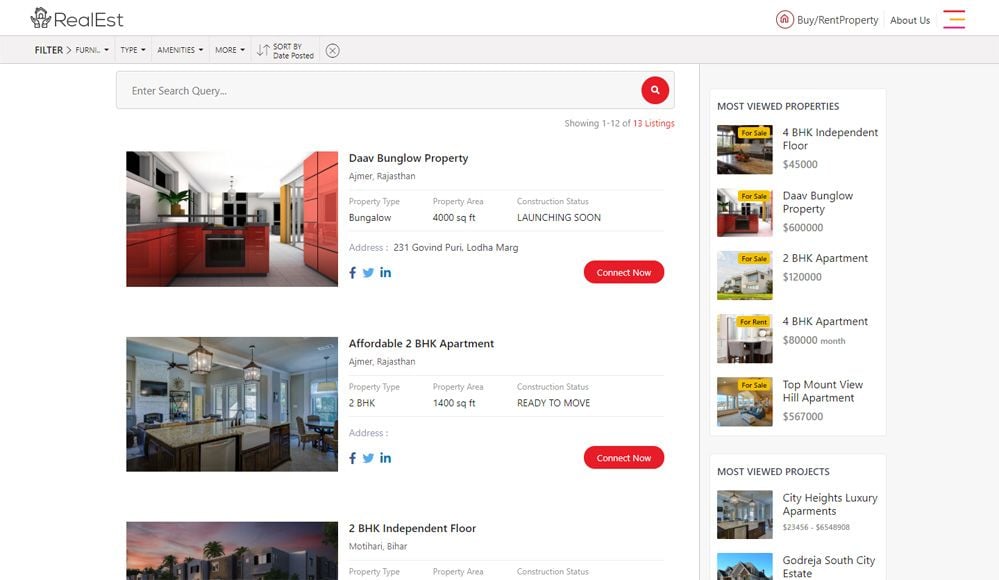This image is a screenshot of a real estate website designed for user-friendly property searches. The website features a prominent logo in the top-left corner that reads "Real EST" in text, accompanied by a logo of a hand holding a house in a drawn style.

On the far-right side of the navigation bar, a series of icons and buttons facilitate user interaction. From left to right, these include a home icon, a circular icon, and text that reads "Buy/Rent Property." Adjacent to this, there's an "About Us" button followed by a distinctive red and yellow hamburger menu, intended to unveil additional settings upon clicking.

Below the main navigation, a banner runs horizontally across the screen, displaying various filter options. These options include "Filter," a right-pointing arrow next to an abbreviation that likely stands for "Furniture," followed by "Type," "Amenities," "More," and finally, "Sort by Date Posted." A circle with an 'X' symbol on the banner suggests these filter options can be modified or removed.

Further down the page, an expansive search bar allows users to input specific criteria for searching properties. This bar features a red magnifying glass icon on its right side. 

Beneath the search bar, the actual property listings are showcased. Each listing includes a small image on the left, accompanied by essential details such as the property's name, address, square footage, and status on the right.

Additional enhancements include social media buttons for Facebook, Twitter, and LinkedIn located at the bottom of each listing, facilitating easy sharing. There is also a prominent red "Connect Now" button in the bottom-right corner of the screen, enabling users to reach out to a realtor for more detailed information on the listed properties.